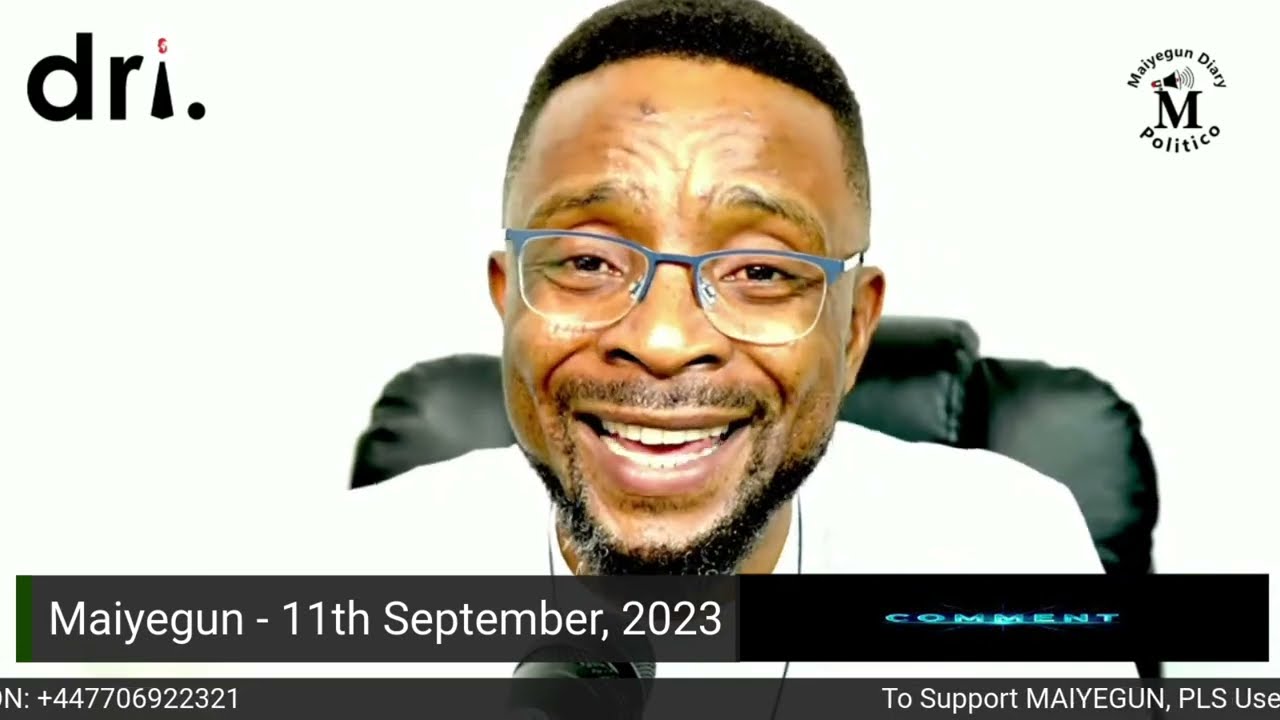The image features a smiling Black man with short hair and bluish-gray glasses positioned high on his face. His bright white teeth are visible behind a beard and goatee, suggesting he was caught mid-sentence or smile. He is sitting in a black leather chair within a white room, speaking into a microphone. Text elements are strewn across the image: "DRI." in black text is in the upper left, while "Myaegon Diary Politico" is in the upper right, with its logo nearby. Below his face, the text "Myaegon 11th September 2023 Comment" is present. The bottom right corner displays a support message: "To support Myaegon please use" followed by a truncated number: "+447706922321." Given the setting and the details, it appears he might be live-streaming from what could be a home office. His slightly squinted, possibly watery eyes add to the emotional intensity of the moment, captured on this particular date.